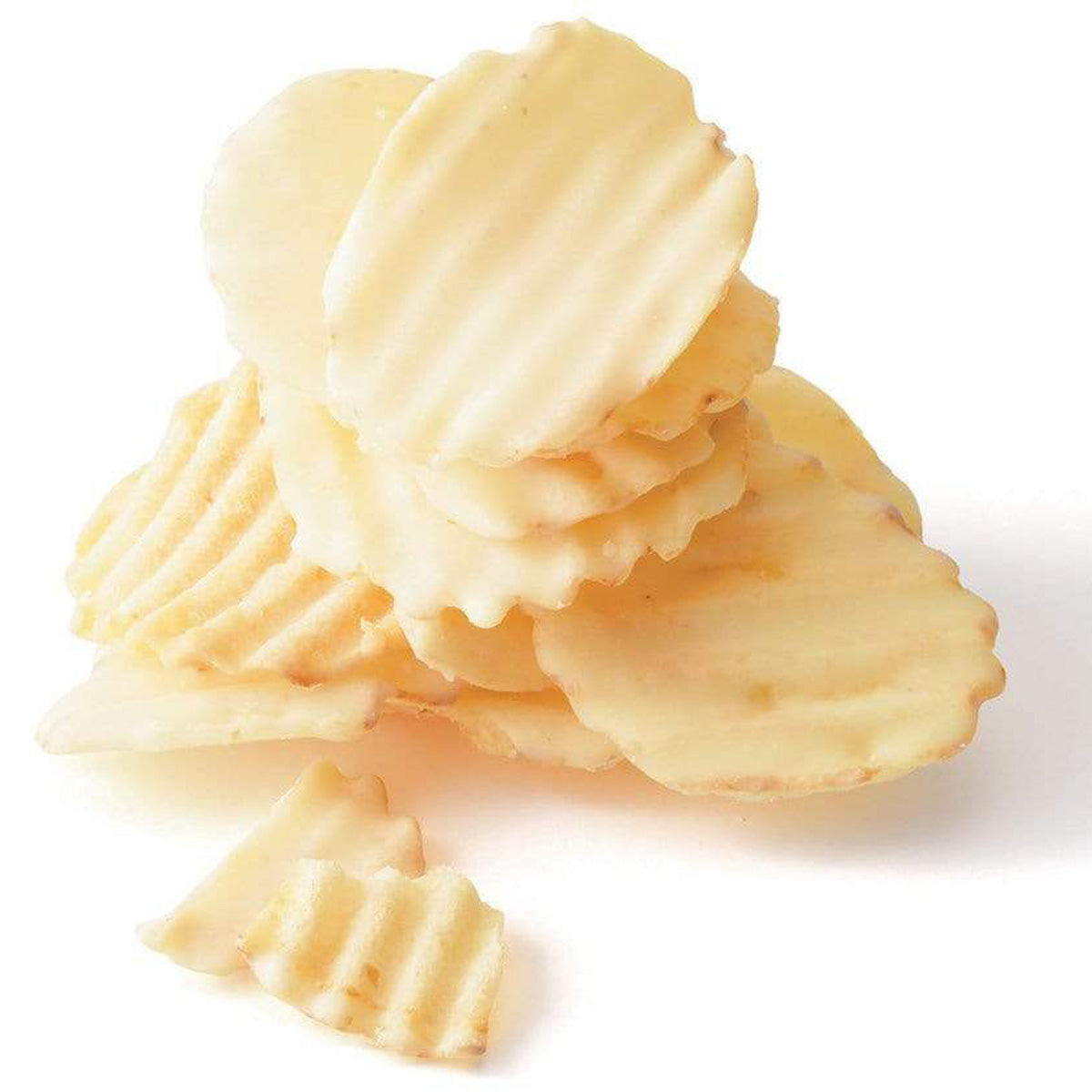This detailed close-up photograph features a stack of golden-colored, ridged potato chips, possibly resembling brand names like Ruffles. The chips are arranged in a rough pyramid shape, with three to four rows tapering upwards into a single stack. Approximately 10 to 11 chips are visible, most of them intact, though there are a few broken pieces near the front of the stack. The photograph is set against a stark white background, with a slight shadow cast to the right, suggesting the light source is from the upper left. The chips appear fresh and crisp, without any visible flavor seasoning, emphasizing their natural appearance.